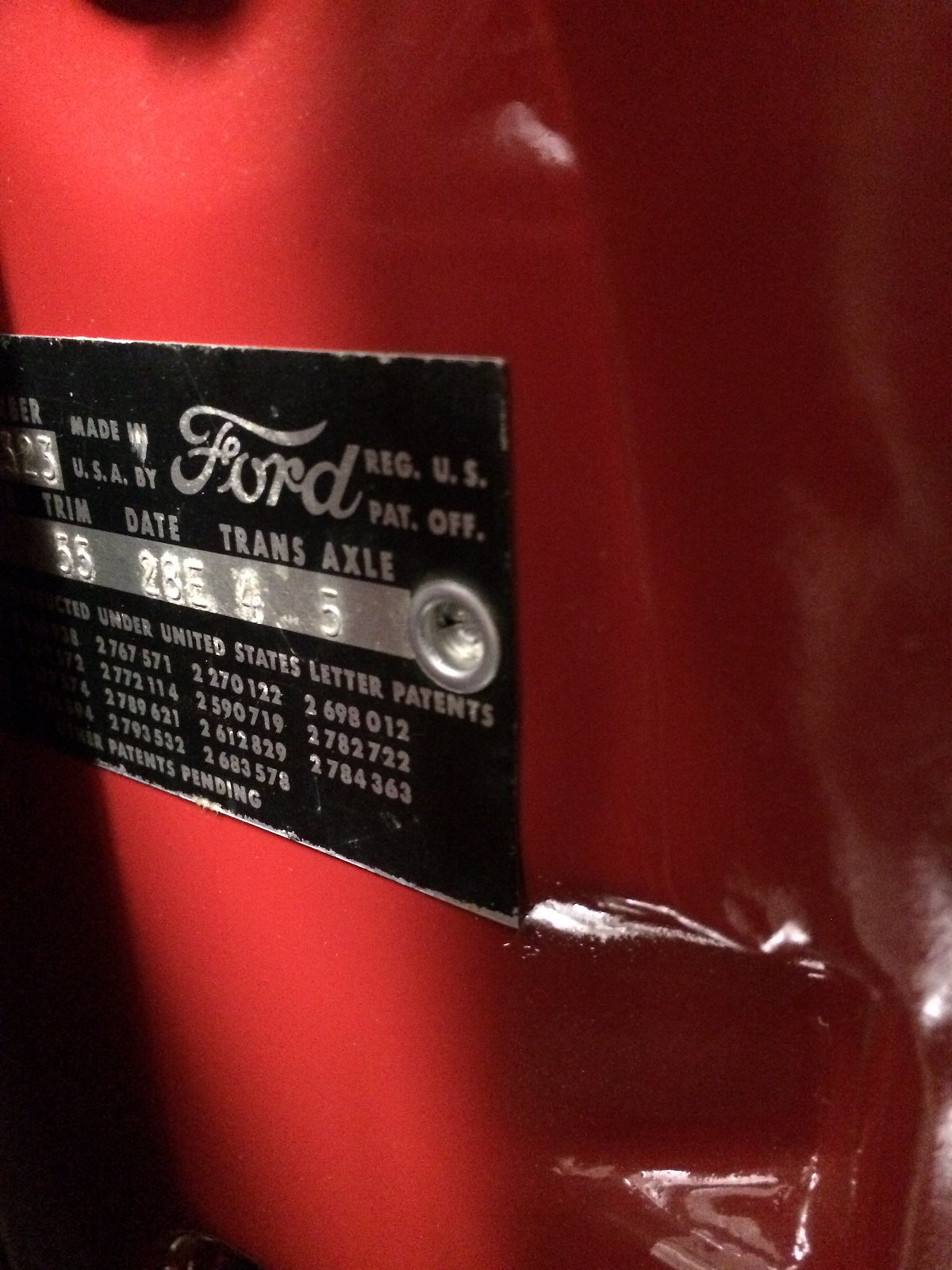A close-up image shows the right section of an older, red metal vehicle, likely a truck, with a small dent crinkling its surface. To the left, there is a black metal patent plate, partially chipped, with the classic Ford logo. The plate includes detailed text such as "Registered U.S. Patent Off", "Trim Date", "Transaxle", and "Made in USA by Ford", alongside multiple patent numbers and a "patent pending" notation. The writing is in silver, and a silver bar runs through the middle of the plate. The metal surface reflects light, evidencing the vehicle's age and rugged use.